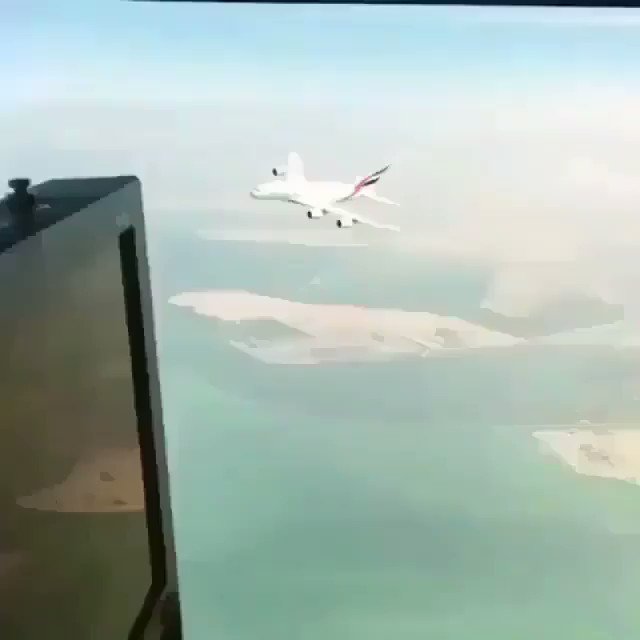In this slightly older, low-resolution image, a white commercial plane is prominently flying high in the sky, centered towards the top. The plane, potentially with four engines—three visible and the fourth hidden underneath—features a logo or colored stripes on its tail rudder. The scenery below is ambiguous, possibly depicting lush green grass with sand pits reminiscent of a golf course or islands surrounded by blue water and beaches. On the left side of the image, there is a black reflective surface, likely part of another plane or building, capturing some reflections from the scene. The image contains no text or additional identifying features.